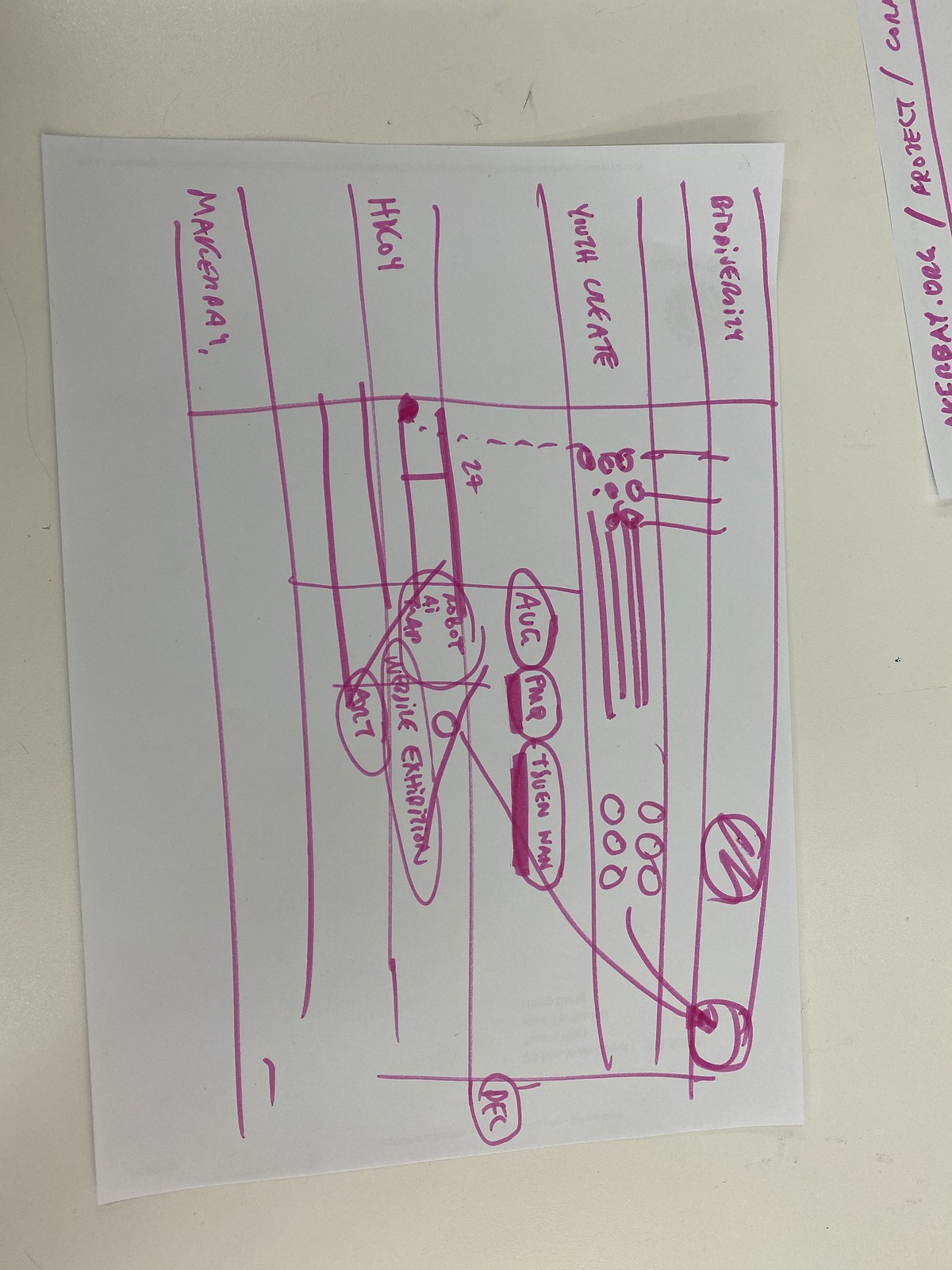A piece of paper is resting on its side atop a dry erase board. At the very top right corner of the board, several words and numbers are visible. The paper itself features a layout with one horizontal line bisecting its width and multiple vertical lines creating columns.

Within the grid formed by these lines, every alternate row starting from the top contains various symbols and text. On the first line, there is a circle with a squiggly line running through it, followed by a second circle with an arrow drawn from the bottom to the top. Skipping a line, the next row contains words accompanied by three small circles, then two circles, and then one circle. Further right on the same line, there are four lines with three sets of circles to the left and three to the right.

The subsequent line is empty with no words, but it does include three circles: two with bold lines drawn underneath and faint, illegible text nearby. Finally, the last row features a circle with a dot inside it, another circle in the form of an oval, and concluding with one simple circle.